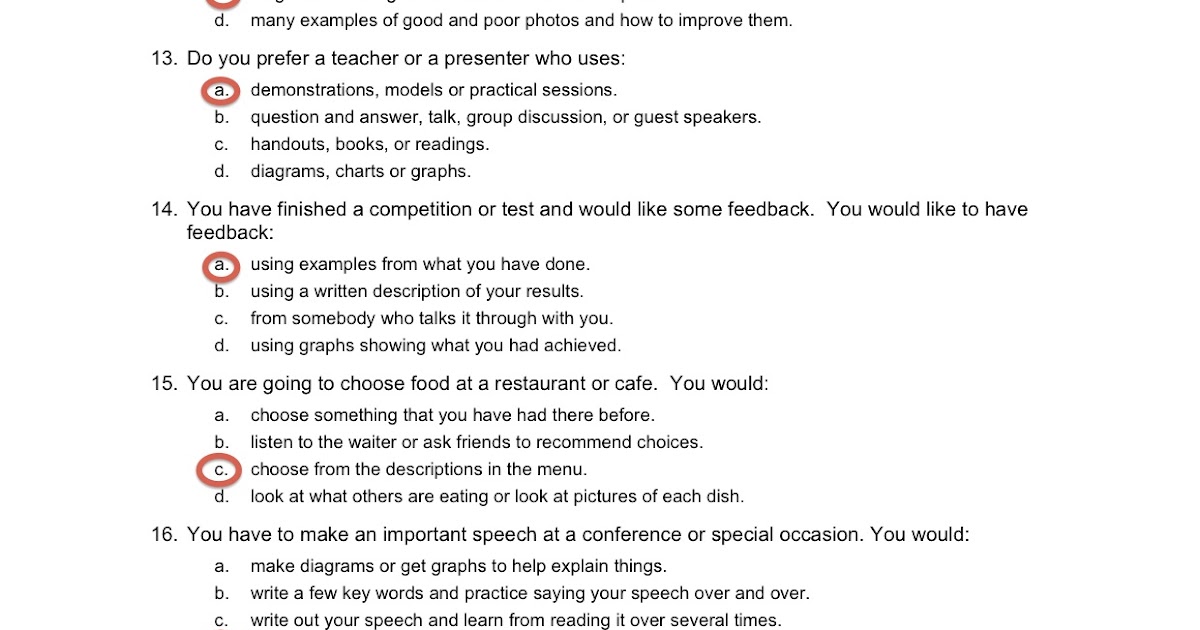This screenshot features a detailed questionnaire formatted in black text on a white background. The layout begins with a section near the top left where there is a bold red circle highlighting the letter "D" followed by a period, and a prompt that reads, "Many examples of good and poor photos and how to improve them."

Further down on the left-hand border, the number "13" appears next to the question, "Do you prefer a teacher or presenter who uses:" with four options labeled A, B, C, and D, each providing different types of instructional methods. The letter "A" is circled in red and corresponds to "Demonstrations, common models, or practical sessions."

Next, at the number "14," the question states, "You have finished a completion or test. Would you like some feedback?" Below this, it continues with, "You would like to have feedback." Below, the options A, B, C, and D are listed with brief descriptions, and once again, the letter "A" is circled in red.

Following this pattern, the number "15" introduces the question: "You are going to choose food at a restaurant or cafe. You would:" with options A through D. This time, the letter "C" is circled in red and accompanied by its corresponding answer.

Finally, at number "16," the last visible question asks, "You have to make an important speech at a press conference or special occasion. You would:" followed by options A, B, and C, but no "D". None of these options are circled red, and the question trails off at the bottom of the screenshot. Each option across all questions includes a brief, one-line response.

This organized layout combines questions with multiple-choice answers, some of which are highlighted with a bold red circle, indicating selected responses.